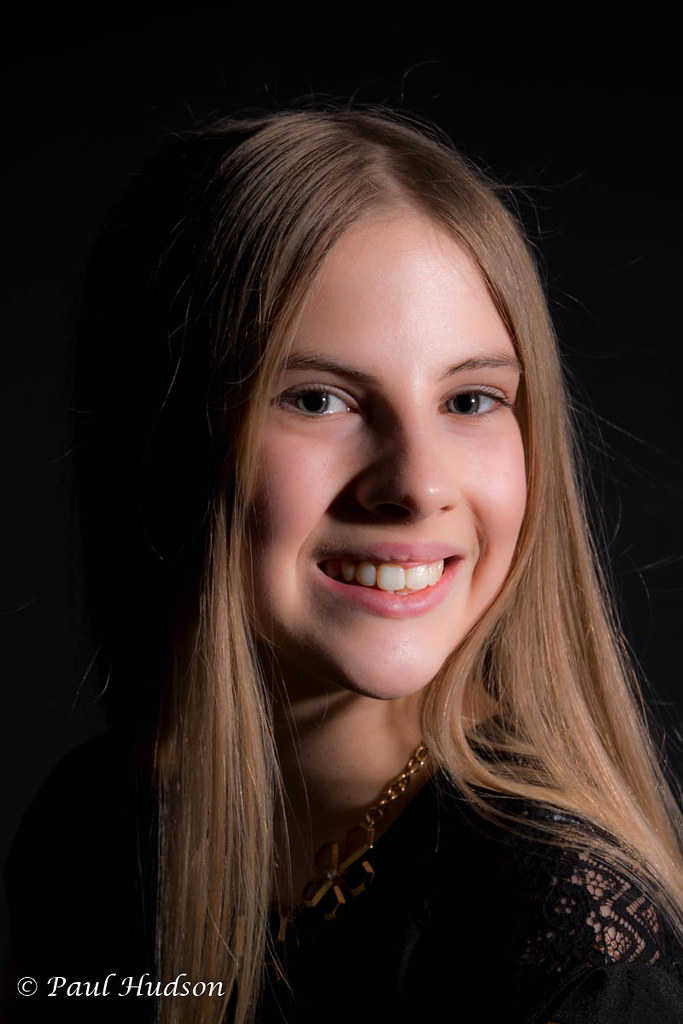This image is a professional headshot of a young woman, likely in her late teens. She has long, blonde hair that cascades down to her shoulders. Her face is illuminated, drawing attention to her big, toothy smile and well-groomed eyebrows. She has hazel eyes and appears to be wearing a subtle amount of makeup. The woman is dressed in a black outfit, accessorized with a gold chain necklace. The background is pitch black, causing her head and hair to gradually fade into it, enhancing the focus on her face. The photograph is professionally lit, suggesting it was taken in a photographer’s studio, possibly for a yearbook or a similar formal purpose. The bottom left corner of the image features the name "Paul Hudson" in white text, indicating the photographer.